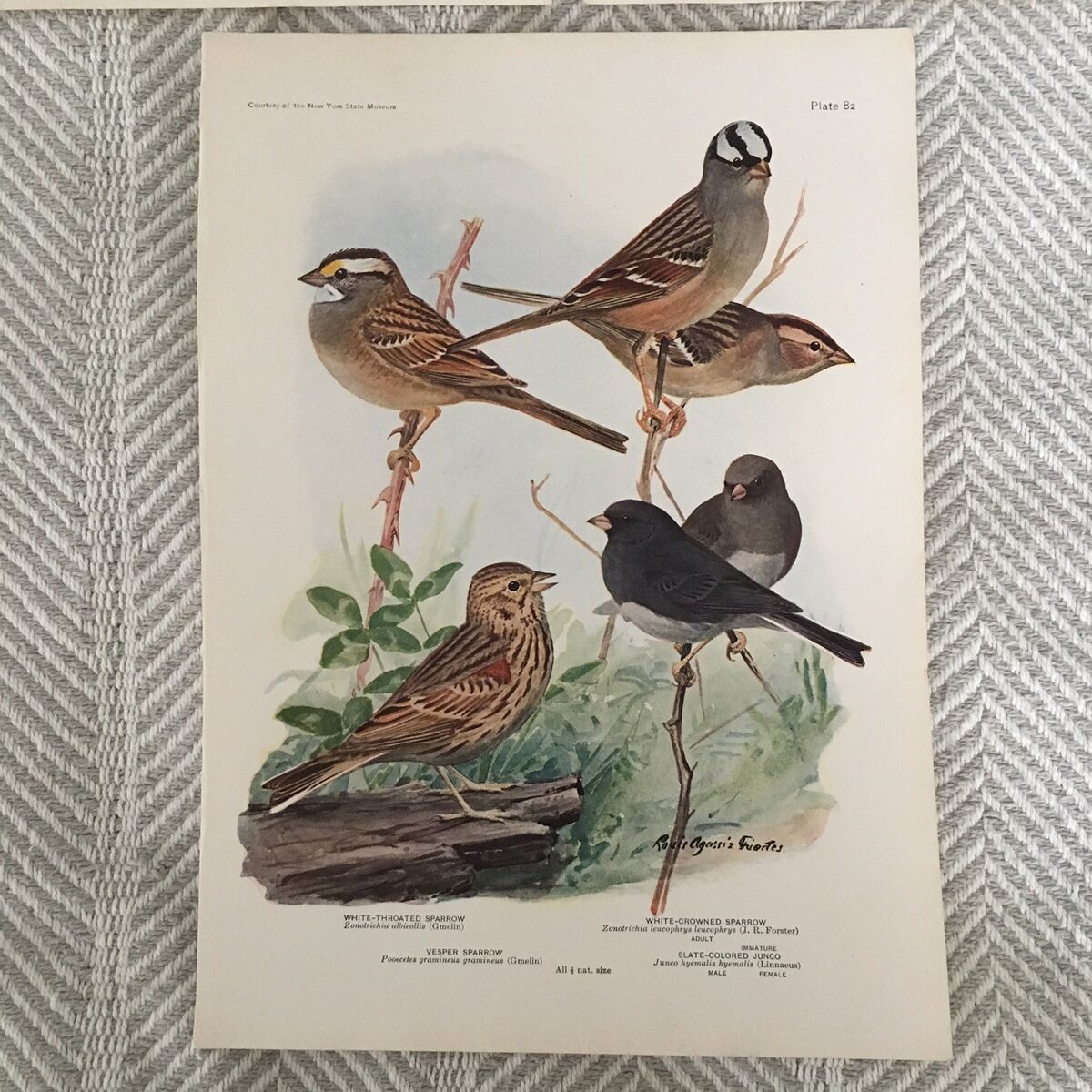This photograph showcases a detailed illustration reminiscent of an Audubon style, though it is signed "Fuentes" at the bottom right. The page, labeled "Plate 82" in the upper right corner and credited to "Courtesy of the New York State Museum" in the upper left, depicts six distinct birds perched on branches and logs with a blue sky backdrop. On a herringbone-patterned fabric, the artwork features three smaller birds at the top with various shades of brown bodies and distinctive black and white striped heads. Below them are two birds with darker bodies—black and deep brown—and white bellies. The lowest bird is characterized by tan and brown stripes and is perched on a small log amidst green vegetation and spiky branches. The bottom of the page has text identifying the birds as follows: "White-throated Sparrow," "Vesper Sparrow," "White-crowned Sparrow," and "Slate-colored Junko," though some of the scientific names are not legible due to focus issues. Notably, it mentions "All NAT Size" in the center, suggesting the birds are depicted in their natural size.